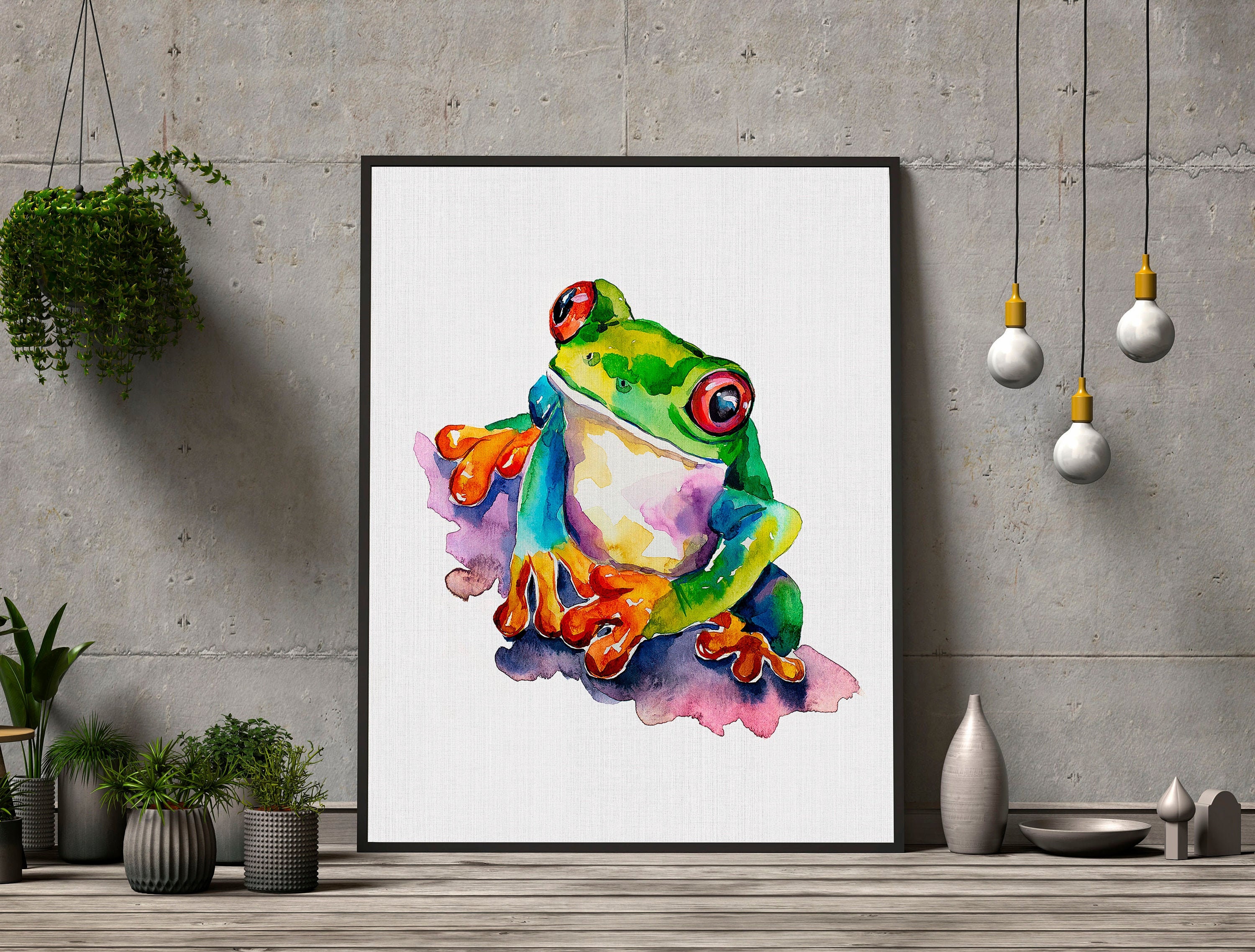The photograph captures a vibrant and artistic scene centered around a large, watercolor-style painting of a frog, prominently displayed against a pitted, gray concrete wall. At the top of the image, a lush fern hangs, with its basket disappearing out of the frame. The painting, leaning on a wooden counter composed of horizontal planks, dominates the center of the image.

The frog in the painting is depicted with a vivid green forehead and back, striking red eyes with black pupils, and teal front legs with orange and red fingers. The frog is perched on a purple and mauve patch, adding context to its pose. Surrounding the painting, to the left, are several small, decorative white pots containing various potted plants, with textures ranging from ridged to bumpy. To the right, empty pots and a bowl complement the setting.

Additionally, three dangling wires with light bulbs at the ends hang on the right side, adding an industrial charm to the space. This eclectic arrangement of plants, decorations, and the colorful frog painting creates a visually captivating and harmonious display.